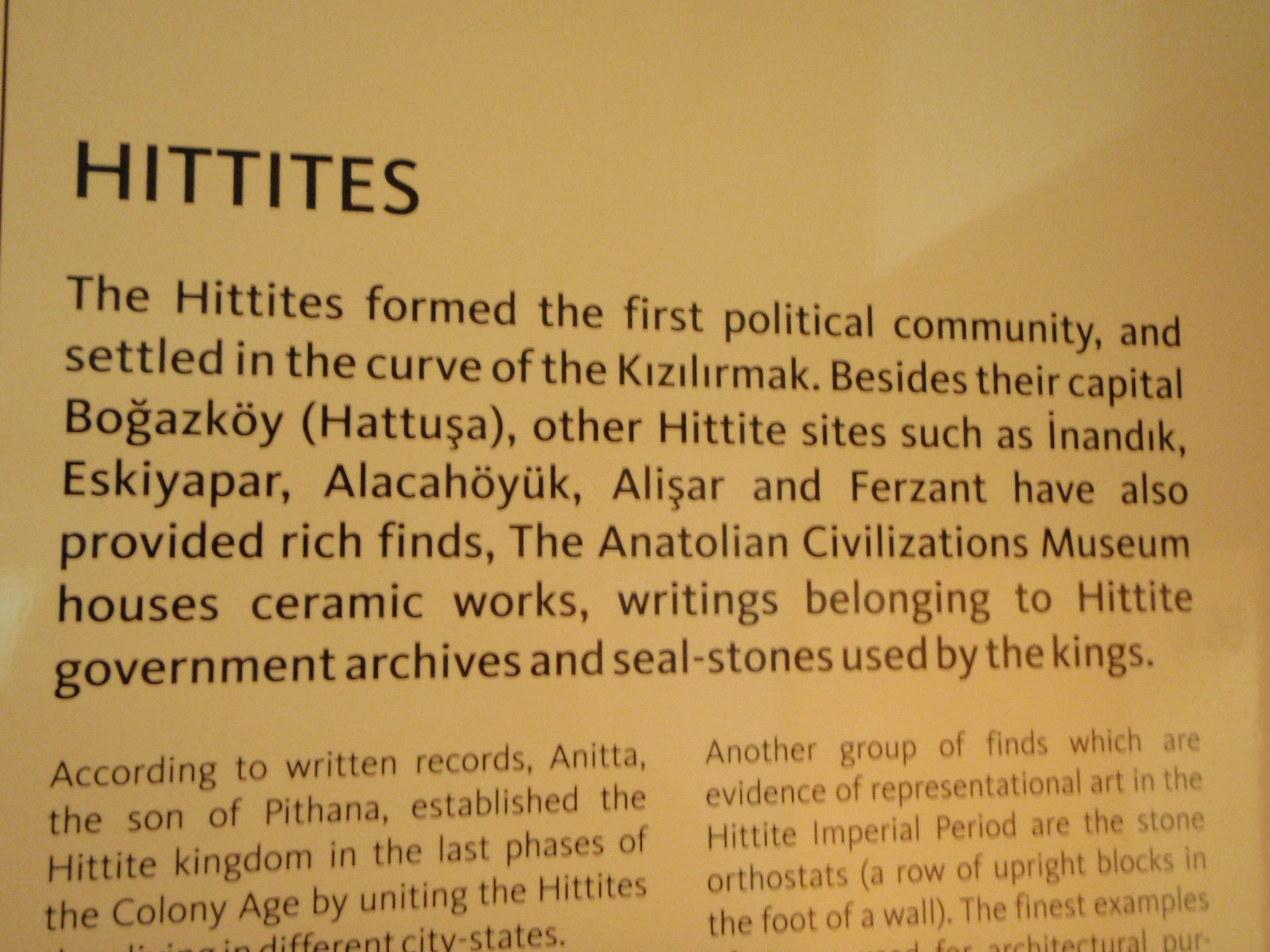The image appears to be either from a book or a museum exhibit, characterized by a background that resembles yellowed paper. The central focus is on a section of text with a white background and black lettering. At the top left, the word "Hittites" is prominently displayed. The main paragraph below details the historical significance of the Hittites, noting that they formed the first political community and settled in the curve of the Kizilirmak River. It highlights their capital, Bogazkoy (also known as Hattusa), and mentions other significant Hittite archaeological sites such as Inandik, Eskiapar, Alacahöyük, Alisar, and Farsan, all of which have yielded rich archaeological findings. Furthermore, it explains that the Anatolian Civilizations Museum houses various artifacts from the Hittite civilization, including ceramic works, governmental writings, archives, and royal seal stones. The bottom of the image features two partially-visible paragraphs, one on the left and one on the right.